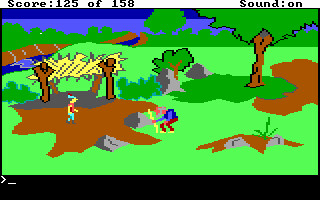This image, reminiscent of an old Atari-style video game, depicts a low-resolution, pixelated scene. At the top-center, a black text overlay reads, "Score: 125 of 158" and "Sound: On." The backdrop features a simplistic blue sky above a green tree line. In the upper left, a brown patch with a blue area underneath symbolizes a river or body of water. Most of the scene is covered in green grass, with a small dirt patch in the bottom left. A yellow banner stretches between two stick-like trees near the dirt patch. 

Standing on the dirt is a small video game character, donned in a green triangular hat, red vest, and blue pants. Adjacent to him, there is an old man with a gray head, wearing a blue shirt and brown pants, holding a yellow walking stick. This old man appears hunched over. The primitive graphics suggest this might be a still from the game "King's Quest," and at the bottom, a DOS prompt is faintly visible, anchoring this retro gaming scene.